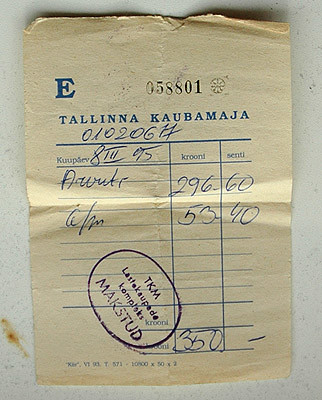This photo depicts an old, worn receipt, yellowed with age and frayed along the edges, likely indicating its age and extensive handling. At the top left corner, there is a prominent, bold blue "E," and to its right, stamped numbers read "058801." The receipt is from the Tallinn Kaubamaja, as indicated by the text. The document details two transactions: one for $296.60 and another for $53.40, summing up to a total of $350, as written at the bottom. Notably, blue ballpoint pen handwriting is visible on the receipt, adding personal annotations or confirmations. The receipt also bears a purple ink stamp, likely official, which partially obscures some text; this might be a notary or certification stamp. The language used on the receipt is not identifiable to the observer, indicating it is not in English.